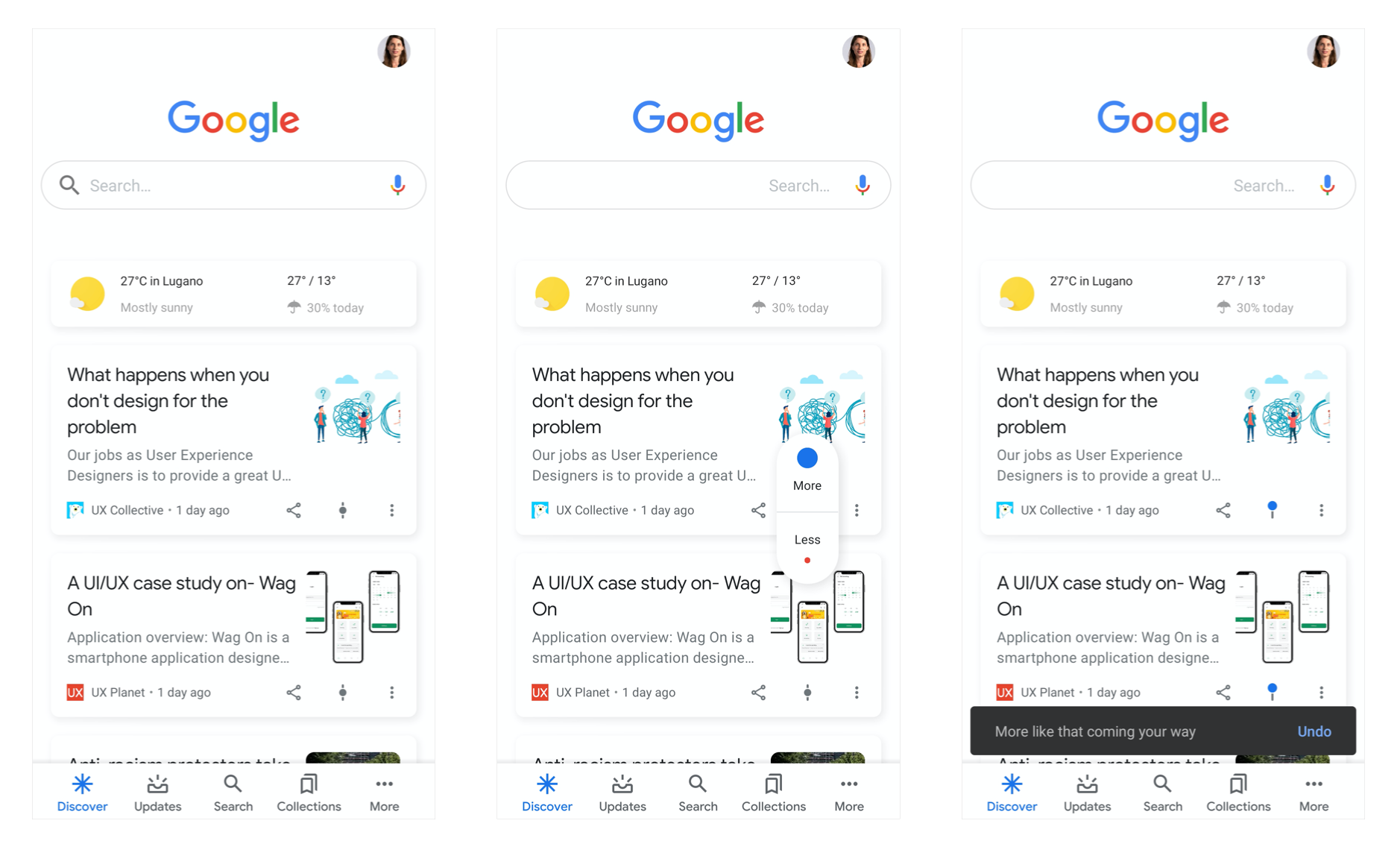This composite image consists of three sequential panels, each depicting a subtle change. In the first panel, located on the far left, a profile photo of a woman with brown hair is positioned in the upper right corner. The center top area prominently features the colorful Google logo in blue, red, yellow, and green, above a standard search bar that includes a microphone icon on the right and a magnifying glass icon on the left.

Below the search bar, weather information for Lugano is displayed, indicating it is mostly sunny at 27 degrees Celsius, with a low of 13 degrees and a 30% chance of rain. Further down, there's a snippet of text discussing the importance of designing for the problem, emphasizing the role of user experience designers (UX) in providing a great user experience (UX collective, posted one day ago). 

Continuing down, the text outlines a UI/UX case study on an application called 'Wagon,' described as a smartphone application designer by UX Planet (posted one day ago). At the bottom of this section, navigation options such as 'Discover,' 'Update,' 'Search,' 'Collections,' and 'More' are listed. To the right, a "More" or "Less" button is visible, with "More" highlighted in blue.

In the final panel on the right, a black pop-up message appears, stating, "More like that coming your way," alongside a blue button labeled "Undo."